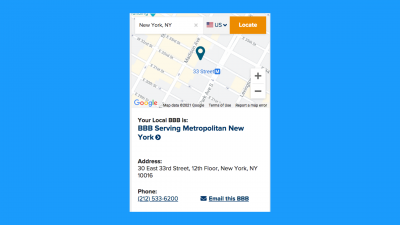The image is a detailed screenshot framed by a prominent blue background. At the center of this background is a screenshot of an application, likely a location or navigation app. 

At the top of the app's interface, there is a white search bar containing the text "New York, NY" in black. To the right, a blue-text button with an American flag icon reads "US," and next to it, an orange button with white text reads "Locate."

Below this top bar, a segment of the Google Map occupies the upper half of the screenshot. A pinpoint marker in aqua is centered on the map. Notable map elements include the Google logo at the bottom left and the text "Map data, Copyright 2021 Google, Terms of Use" at the bottom right. Adjacent to this text is some unreadable information. On the right side of the map, a vertical zoom control featuring plus and minus signs is visible. Directly beneath the pinpoint marker is a partially visible "M" icon next to an unreadable blue text label.

The lower half of the screenshot shifts to an informational section. It starts with black text that reads, "Your local [unreadable] is," followed by bolder blue text stating, "888 serving Metropolitan New York," accompanied by a blue arrow. 

Further down, the address details are provided in fine black text: "Address, 30 East, 33rd Street, 12th Floor, New York, NY 10016." Below this, bold black text labeled "Phone" is followed by a thinner blue text displaying the number, "212-533-6200," positioned towards the bottom left.

Finally, at the bottom right corner, another bold text with an email icon states, "Email this 888."